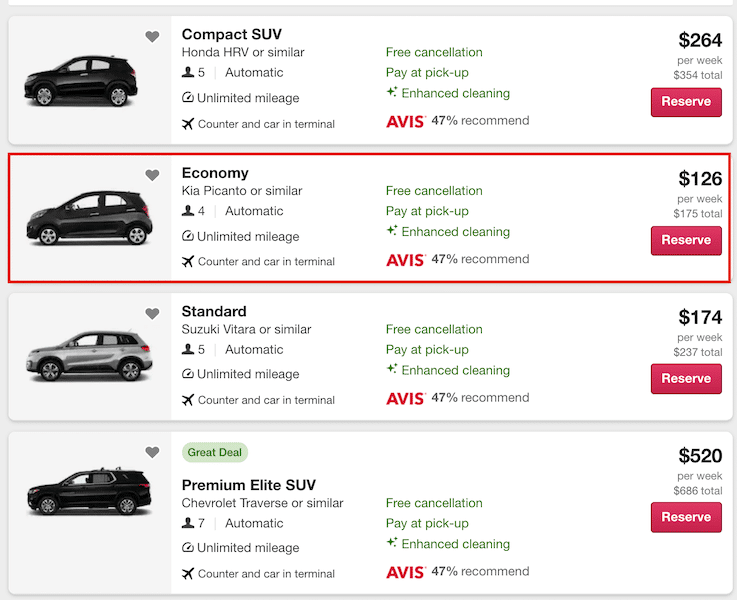This image showcases four vehicles available for rental from Avis Car Rental Company, displayed on elongated rectangular cards arranged vertically. Each card provides detailed information about a specific vehicle. The second card from the top highlights a vehicle, outlined in red, drawing immediate attention. The vehicles presented include:

1. **Compact SUV:** Honda HR-V or similar
2. **Economy Car:** Kia Picanto or similar
3. **Standard SUV:** Suzuki Vitara or similar
4. **Premium Elite SUV:** Chevrolet Traverse or similar

For each vehicle, the cards detail essential information such as unlimited mileage availability, seating capacity, transmission type (automatic or manual), and pickup locations (whether at the counter or in-terminal). Additionally, each card features a "Reserve" button as a call to action for potential renters. The cards also display a percentage recommendation for each vehicle, providing renters with customer satisfaction insights.